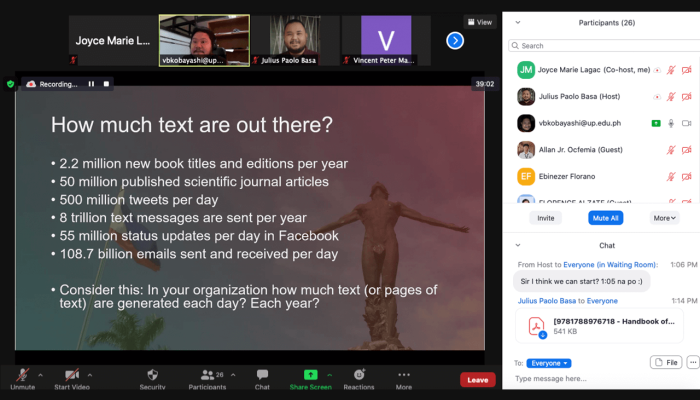The image features a predominantly black background at the top, where a series of smaller images are arranged. Starting from the left, the first image displays the text "Joyce Marie L" followed by an ellipsis (…). Adjacent to this is an image of a man with short black hair, standing in front of a shelf. His username is displayed beneath his image as "vbkobzyash," followed by an ellipsis (…). Next to him is another individual with short hair, a short beard, and a mustache, wearing a burgundy shirt. His name is given as "Julius Polo," with additional text reading "B/15-1."

Continuing to the right, there is an image with a purple background and a white "V" in the center, labeled "Vincent Peter." The name is partially cut off, showing only the first letters "MA." Additionally, a circular icon with a blue arrow is present. Towards the bottom right corner, the number "39.02" is displayed.

There is also a banner or pop-up featured in the image. This pop-up poses a question, "How much texts are out there?" and includes a description urging viewers to "consider this: in your organization, how much text or pages of text are generated each day, each year?" On the right side of the screen, there is a section labeled "Participants," listing usernames and offering options to "invite," "mute all," or explore "more."